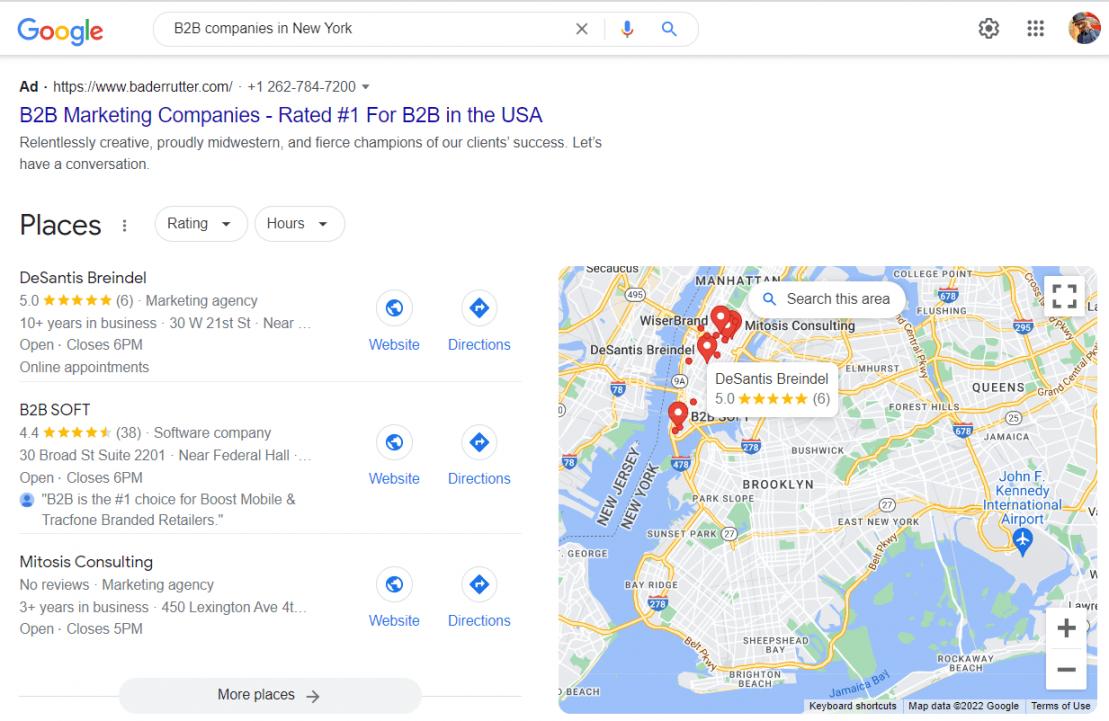The image depicts a Google search results page for the query "B2B companies in New York." At the top left corner, the Google logo is prominent, followed by a search bar where the query has been entered. Below the search bar is a highlighted snippet in purple text that reads "B2B marketing companies rated number one for B2B in the USA."

The search results list begins with DeSantis Braindell, which offers online appointments, has been in business for 10 years, and has a five-star rating. Following that is B2B Soft, which boasts nearly a five-star rating, is located on Broad Street, and is noted as the number one choice for Boost Mobile and Tracfone branded retailers. Mitosis Consulting is also listed; it has been in business for three years but currently has no reviews and is situated on Lexington Avenue.

On the right side of the page, there is a map highlighting parts of New York, including Manhattan, Brooklyn, Queens, and a portion of Staten Island, as well as part of New Jersey. Someone has drawn in red on the map, featuring circles and red dots, with one circle vaguely resembling the letter "B."